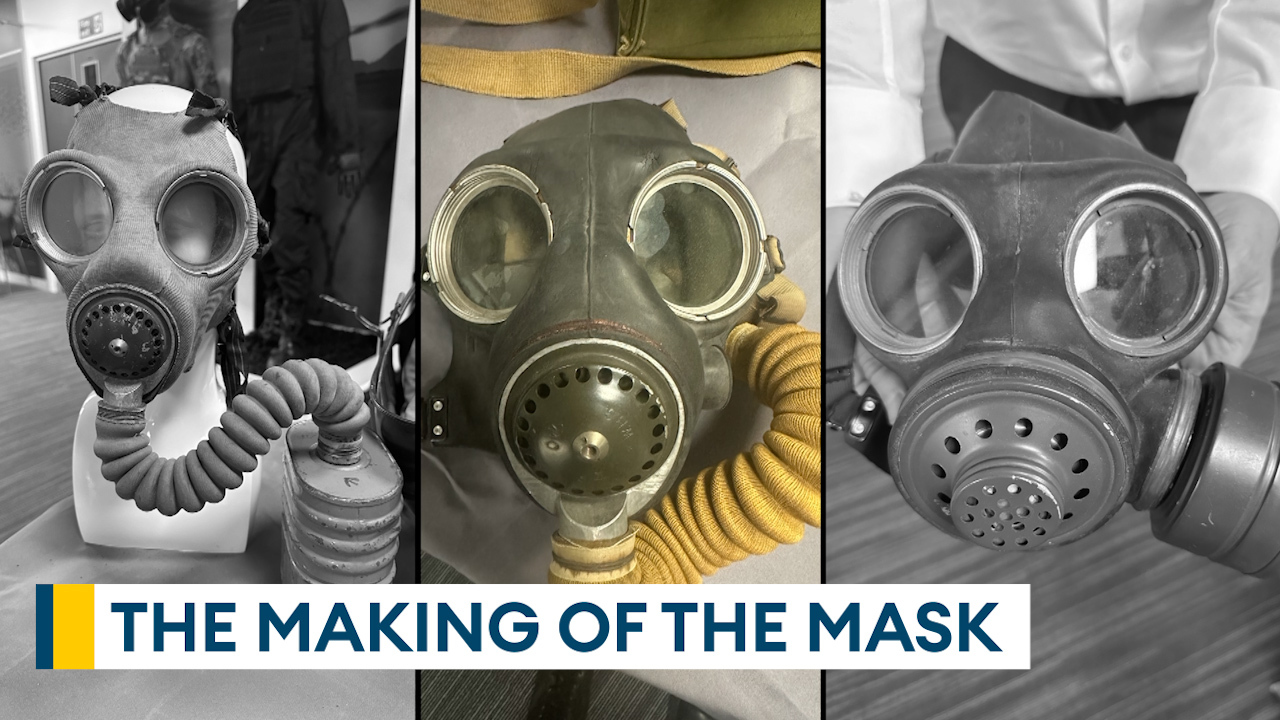The image titled "The Making of the Mask" is a poster divided into three side-by-side sections, illustrating the evolution of gas masks through detailed vintage portrayals. Each section features a different style of gas mask, all of which are visually distinctive and representative of World War II era equipment. The first and third images are in black and white, while the second is colorized, highlighting the contrast in design and materials.

The first gas mask, mounted on a dummy's head, is equipped with a metal respirator and two round glass eye holes. It is connected to a silver canister via a coiled tube. The second gas mask, depicted in olive green, features a fabric coiled tube that hooks into the side, integrating with the respirator. The third gas mask, also with round glass eyes and a metal respirator, has a canister attached to the side of the face.

A white banner with blue and yellow markings spans across the image, bearing the title "The Making of the Mask" in blue letters. This comprehensive layout provides a visual narrative of the incremental improvements in gas mask designs, each subsequent mask featuring enhancements over its predecessors. Large circular eye pieces and breathing filters are consistent design elements across all three masks, showcasing the essential features needed for effective protection during wartime.